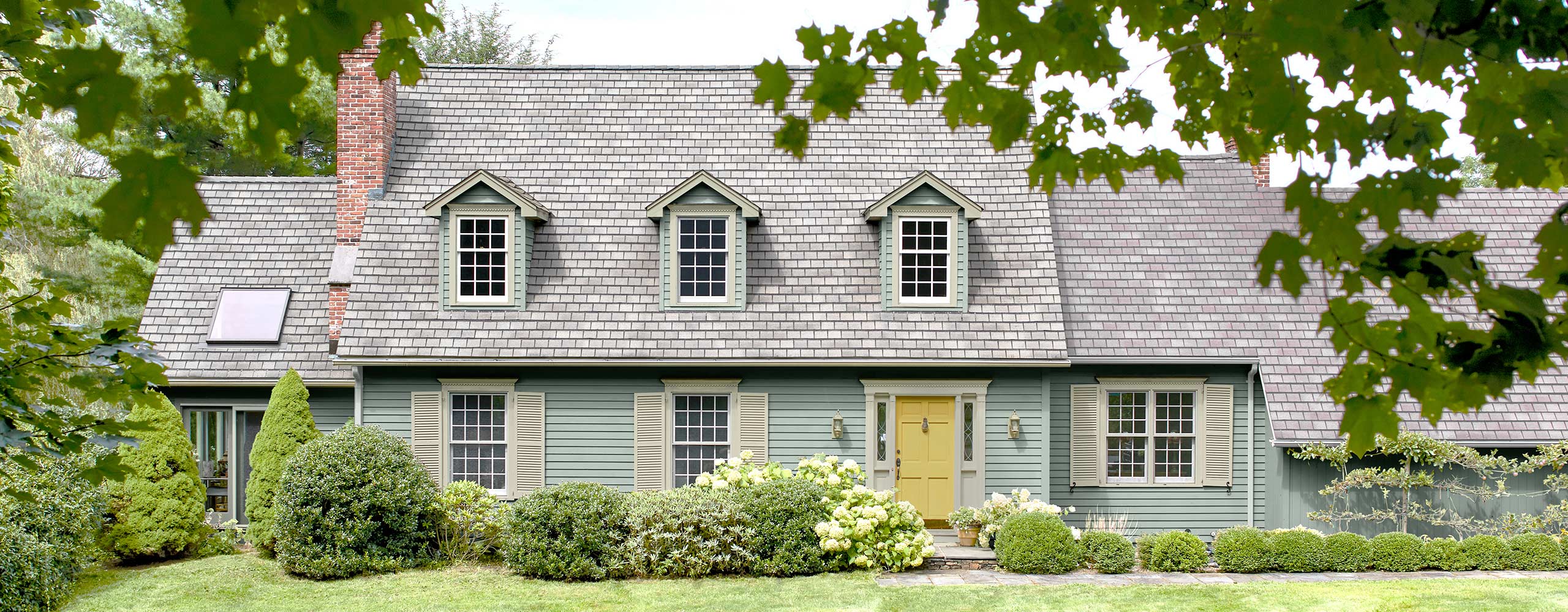This photograph captures a serene and picturesque scene of a beautiful, expansive home that exudes an almost ethereal, computer-generated quality due to its immaculate appearance. The house features light turquoise or sage green siding, highlighted by a striking bright yellow front door flanked by two side lights and adorned with tan shutters on the first-floor windows. The roof is light gray and has three charming dormer windows, along with a skylight. The home boasts a large, well-manicured lawn surrounded by vibrant green trees, ornate flower beds, and neat landscaping that includes small green bushes and white hydrangeas near the entrance.

To the left of the house, there is a pink brick chimney which suggests the presence of a cozy brick fireplace indoors. Adjacent to this chimney is an enclosed sunroom. On the right side of the house, which extends possibly to an attached garage, the structure seems to be larger than initially perceived, suggesting ample living space. The photograph also captures branches and blurred oak leaves from a tree in the top corners, adding a natural frame and emphasizing the tranquility of the scene. The sky is covered with gray clouds, contributing to the peaceful and serene ambiance, reminiscent of a calm spring or summer day.